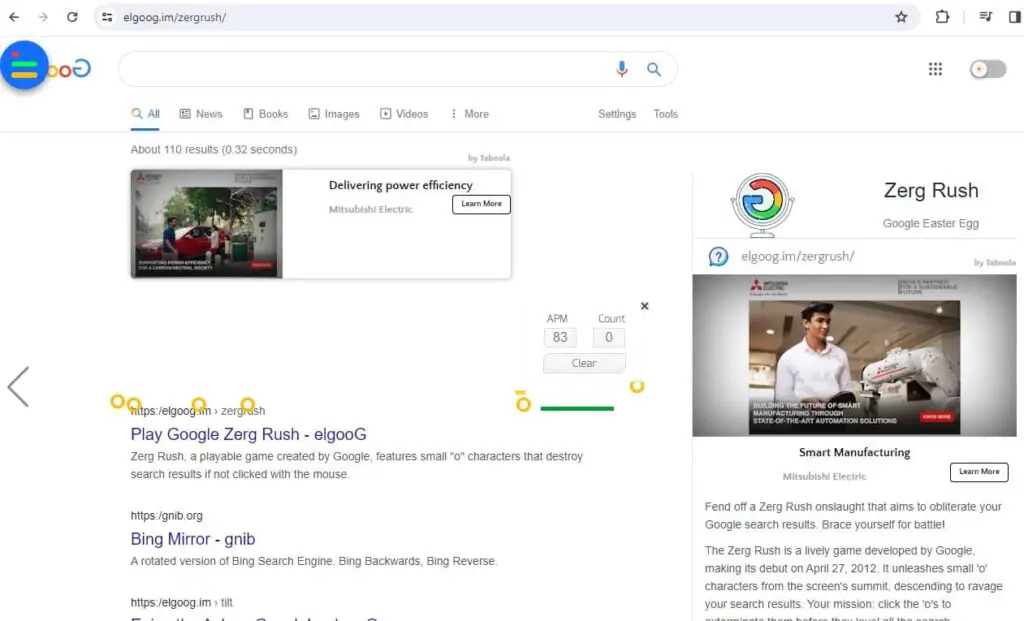**Detailed Caption:**

The image showcases a Google search page with the URL "elgoog.im/zcrash" displayed at the top, written in reverse. The Google icon in the top left corner is also mirrored. The search results page is presented with the characteristic Google colors: blue, green, yellow, and red, though reversed. At the bottom, it indicates approximately 110 results were found in 0.32 seconds.

Below this, there is an advertisement on the right side promoting Mitsubishi Electric with the text "Delivering Power Efficiency - Mitsubishi Electric. Learn More." Underneath this ad, the Google URL is again reversed, and it reads "play cookie cookie zcrash." This references a game called Zcrash, created by Cookie, where small characters appear on the search results and must be clicked with the mouse to prevent them from causing destruction. Yellow circles, which are part of the game, appear at the bottom of the screen.

Another URL, also mirrored, reads "bing mirror GNIP," denoting a reversed version of the Bing search engine. To the right, it emphasizes the Zcrash game, with the letter "G" facing in the opposite direction. Further details state, "Start Manufacturing Mitsubishi Electric - Fend off Zcrash onslaught that aims to obliterate search results. Brace yourself for the battle." 

Zcrash is described as a vibrant game created by Cookie, launching on April 27, 2012. The game involves small characters descending from the top of the screen to attack search results, and the player must click the "O"s to stop them from causing chaos.